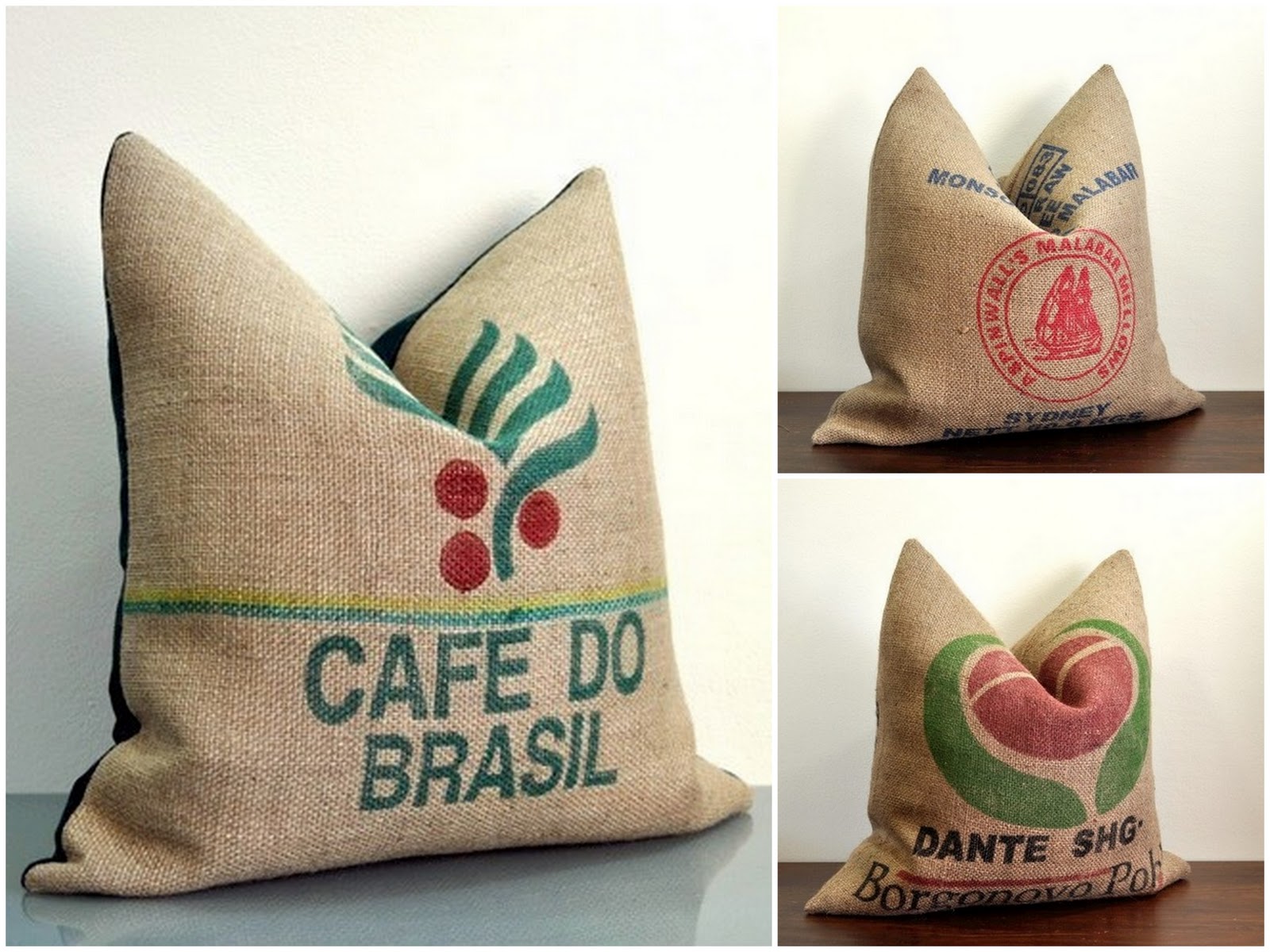This image presents a vertically oriented, rectangular grid featuring three separate photos of burlap sacks, commonly used for storing coffee. The left half of the image showcases a single, larger burlap bag placed on a surface that appears shiny and greenish-gray, against a white wall background. This bag is tan with green and yellow stripes and bears the text "Café do Brasil." Above the text is a green and red design resembling a plant with berries.

The right half of the image is divided into two smaller, square pictures. The top picture displays another burlap sack on a wooden floor, featuring blue text and a depiction of a sailing ship with red text that reads "Aspen Walls Malabar Mellows." Below, there is another burlap sack on a similar wooden surface. This bag displays a red and green logo with black text stating "Dante S.H.G."

All three sacks share a similar color palette and coarse material, and each displays unique branding and logos, providing a cohesive yet varied collection of burlap coffee bags.